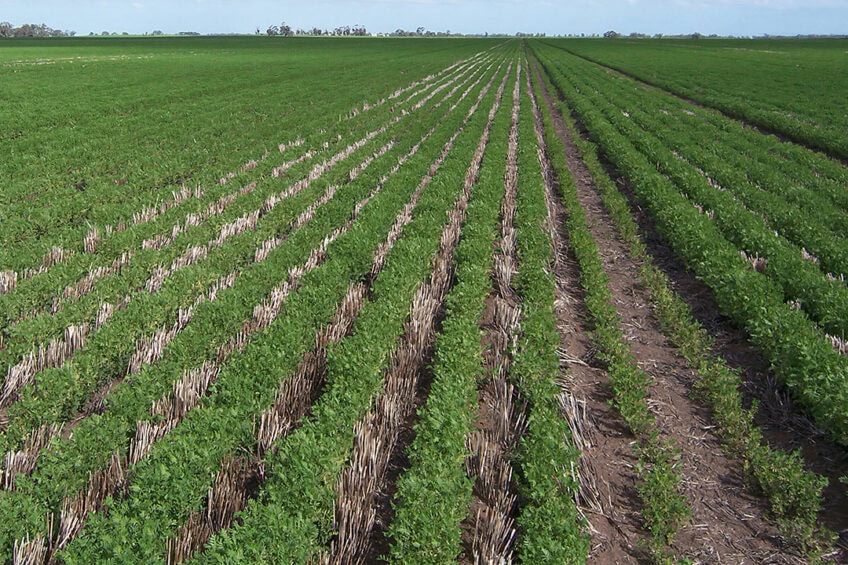This is a detailed horizontal color photograph of a vast farmland, likely part of a large agricultural area. The perspective from the vantage point reveals alternating rows of green leafy plants, approximately six inches wide, and brown rows of either dirt or dried grass and sticks, stretching from the foreground into the distance. These rows converge towards a central point, indicating meticulous planting patterns across acres of land. The crops appear recently planted, as there are no visibly blooming plants yet. The background is characterized by a flat, empty horizon with very few buildings and small patches of trees dotting the landscape. Beyond the farmland, the view extends to distant hills under a clear, blue sky devoid of clouds, creating a serene and expansive rural scene.